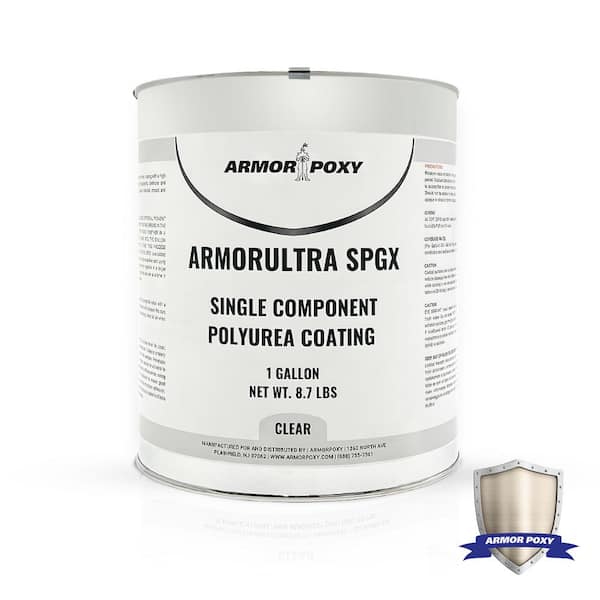The image depicts a silver and white bucket, reminiscent of a paint can, used for containing a coating product. The bucket features a prominent white label with multiple lines of descriptive text in black. At the top of the label, within a white semicircle bordered by a black outline, it reads "ArmorProxy". Directly below that, it states "Armor Ultra SPGX," followed by "single component polyurea coating." Further down, the label specifies "one gallon, net weight 8.7 pounds" and "clear," with the word "clear" uniquely presented on a silver banner against the white background. Positioned at the bottom right of the image is a silver shield graphic, adorned with rivet head details around its edge and the words "ArmorProxy" inscribed on it. The overall product design emphasizes its high-quality construction and detailed labeling.